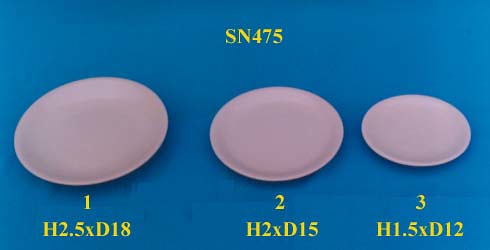The image features a mid-shade blue background with the text "SN475" printed in yellow at the top. Below this, there are three light grayish-pink circular shapes of varying sizes arranged from left to right, largest to smallest. Each circle has a thin edge that thickens slightly toward the center. The left circle, the largest, has the label "H2.5 x D18" in yellow text beneath it. The middle circle, slightly smaller, is labeled "H2 x D15." The right circle, the smallest, is marked with "H1.5 x D12."